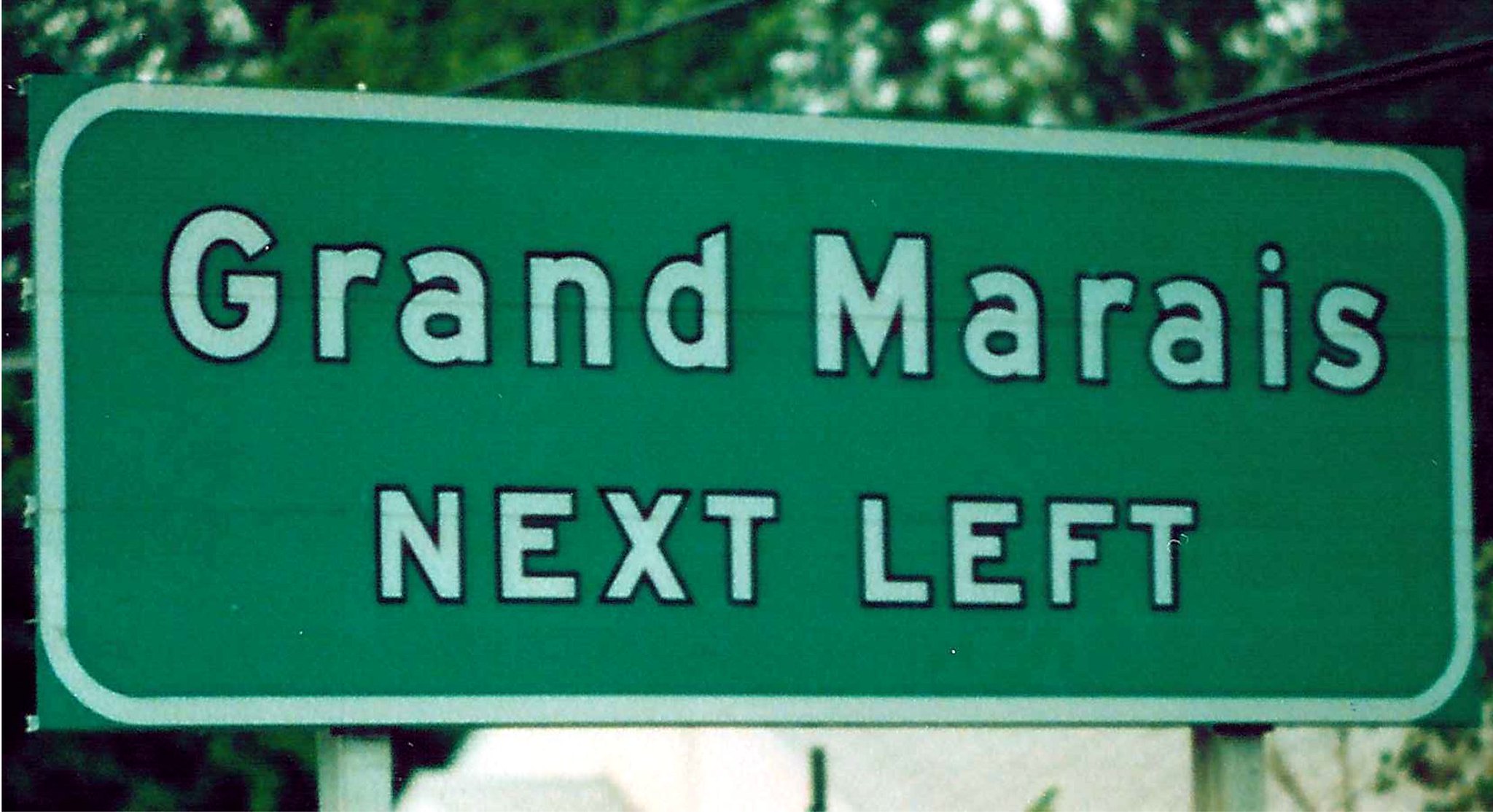This horizontal image, with dimensions twice as wide as it is tall, prominently features a street sign that occupies the entire frame. The sign is green, bordered in white, and displays text in both uppercase and lowercase letters, all white with black outlines. The upper portion reads "Grand Marius," while the bottom line, in all caps, declares "NEXT LEFT." The sign is affixed to two square metal posts. In the background, a network of power lines crisscrosses the scene, interspersed with abundant green trees. A light sky peeks through the foliage, and a white building is partially visible beneath the sign, adding depth to the urban landscape.